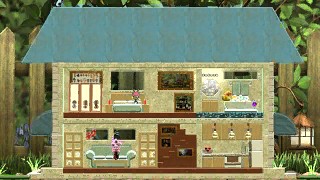The image depicts a charming dollhouse captured from a distance, showcasing both its intricate exterior and detailed interior. The roof of the dollhouse is a vibrant blue, easily catching the eye. Inside, the cozy layout includes a bedroom on the left, where a neatly made bed is visible. On the right side, a pristine white bathtub stands out. Directly below this, the kitchen area is illuminated by three lights and outfitted with miniature appliances and fixtures, emphasizing the dollhouse's attention to detail. 

On the far left, a figure is positioned atop a blue couch, adding a touch of life and activity to the scene. Surrounding the dollhouse, various blades of grass and plants create a lush, natural environment, while a white and beige tall fence encloses the background, harmoniously matching the dollhouse’s color palette. The picture exquisitely blends the whimsical charm of the dollhouse with the serenity of the outdoor setting.